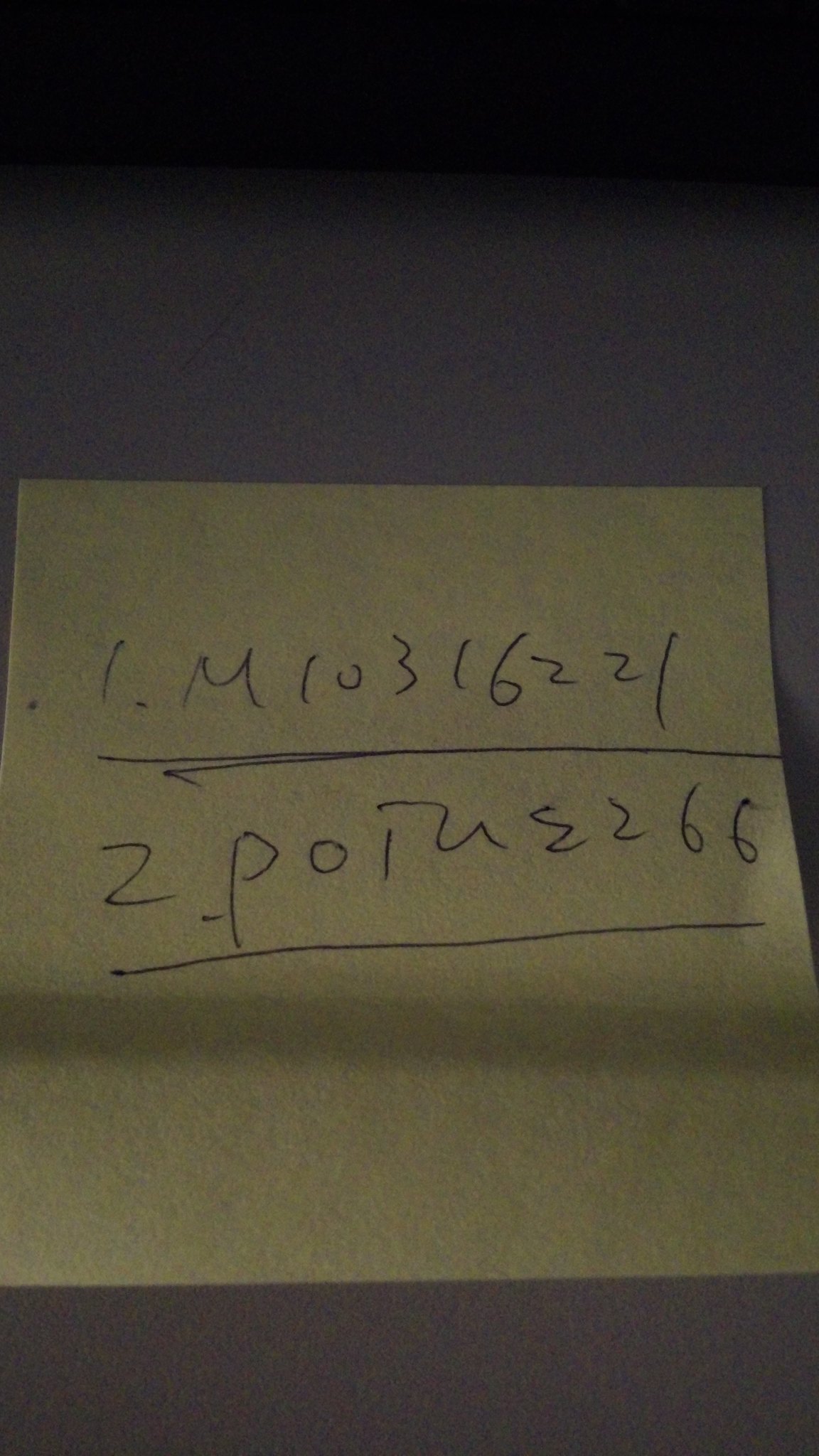The photograph captures a somewhat dark and shadowy scene where a square sticky note, commonly known as a post-it note, is prominently adhered to what appears to be the edge of a tabletop. The tabletop extends about two-thirds down the sticky note, causing the remaining third to fold over the edge, creating a natural bend. The sticky note is positioned such that it appears to hang off a small shelf formed by the table's edge. 

The sticky note itself is a pale yellow color and features two handwritten entries, both written in black ink. The first entry, labeled with the number "1," reads "M10316221" and is underscored with a solid black line. Under this entry, the second item, labeled with the number "2," reads "POTUE266," also underscored with a black line. The writing is clear and orderly, indicative of a deliberate and precise note-taking process.

The background, including the tabletop, is predominantly dark, making it difficult to discern the exact color and details of the table. The surface appears to be either medium gray or medium brown, but its exact hue is obscured by the low lighting. The focus of the composition is entirely on the sticky note and its written content, which stands out starkly against the gloomy backdrop.